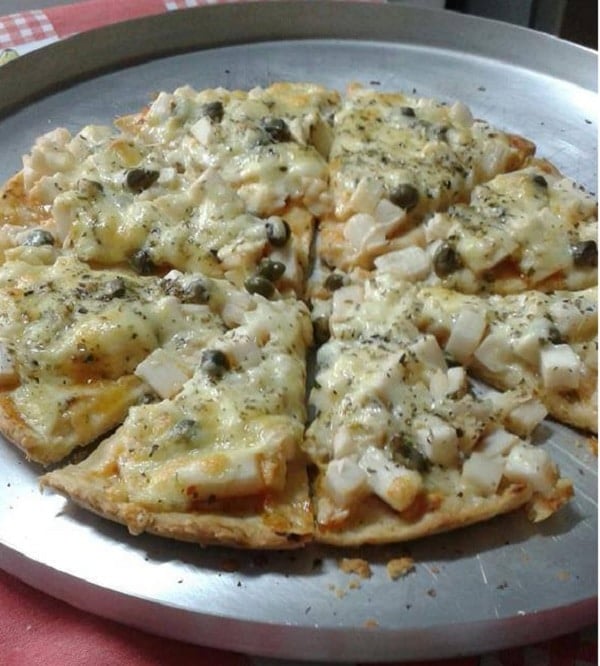Here's a detailed caption combining the shared and repeated elements from the three descriptions:

In this close-up image, a custom-made thin-crust pizza rests on a silver-colored metal pan, likely made of aluminum. The pizza is cut into eight slices and sits atop a red and white tablecloth. The crust is very thin, suggesting a flatbread-style pizza. The toppings include melted white cheese, squares of brown-crusted potatoes, and sliced black olives. Additionally, specks of a green spice, possibly oregano or pepper, are scattered across the top. There are a few crumbs visible on the front and back sides of the crust. The pizza does not appear to have any tomato sauce, and the overall presentation is enhanced by the contrasting tablecloth underneath.